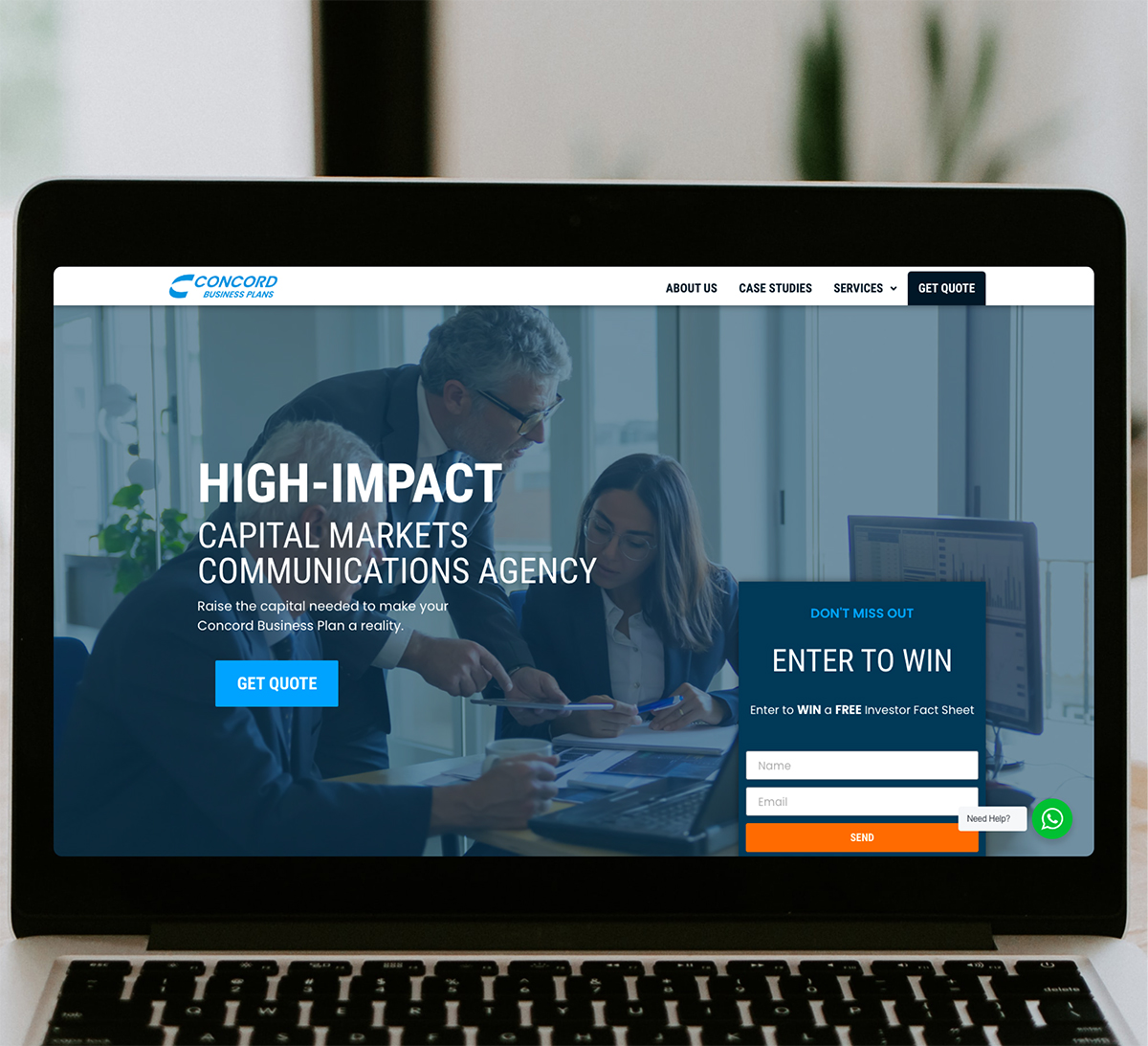A close-up view of an open laptop computer reveals a detailed shot of the upper part of the keyboard and the screen. The keyboard itself features black keys set against a silvery-gray keyboard pad, showcasing a sleek design. The screen displays a website identified by the text "Concord Business Plans" prominently located in the upper left corner. 

Further details include navigation links such as "About Us," "Case Studies," "Services," and "Get in Touch," written in white text on a black rectangular bar in the upper right corner. The main content on the screen shows a large image featuring three individuals; two are seated at a table, while one stands, all engaged in reviewing documents. They are dressed in professional black and white attire, suggesting a formal business setting. 

Additionally, in the right section of the screen, white text on a dark blue background reads "Enter to Win." The overall composition highlights the professional and organized layout of the website displayed on the laptop.